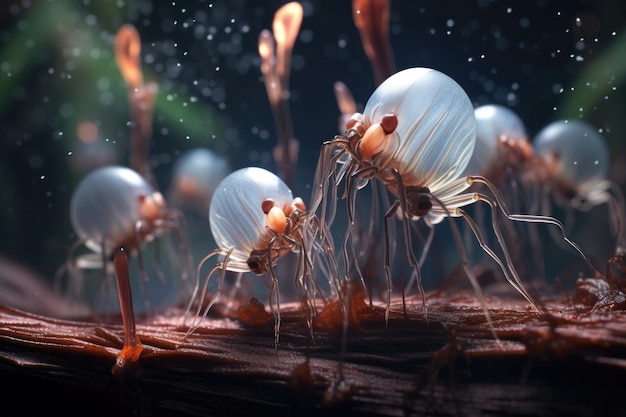This is a detailed 3D render of water fleas, depicted in a close-up, underwater scene. Two water fleas are prominently in focus near the center, one slightly smaller than the other, while several more appear blurred in the background. The fleas sport white, bulbous bodies adorned with more than a dozen slender, gray legs. Each of their heads features a striking red circle atop an orange stalk, which adds a touch of vivid color to their transparent forms. The creatures appear to be standing or walking on a floating object, possibly a piece of wood or organic debris.

The image, in landscape orientation, captures the underwater ambiance with a reddish-brown textured surface below, reminiscent of the ocean floor. The backdrop is predominantly dark, punctuated by floating white particles and out-of-focus, orange stalk-like formations. Despite being a render, the image achieves a level of realism that makes the water fleas' intricate details and their spider-like, jellyfish qualities stand out. The composition and reflective elements of the render evoke a fantastical scene, almost as if these fascinating creatures are walking by a mirror in an underwater world.